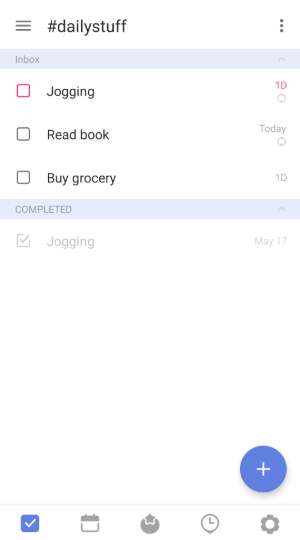The image displays a mobile app interface named "DailyStuff," designed for activity tracking. The screen is divided into sections labeled "Inbox" and "Completed." Within the "Inbox," there are three tasks: "jogging," "read book," and "buy grocery," each accompanied by an unchecked checkbox. In the "Completed" section, there's the task "jogging" with a checkmark beside it, indicating it was finished on May 17. The other tasks in the "Inbox" are presumably for today and lack specified dates. The background of the app is predominantly white, creating a clean and simple aesthetic. At the bottom of the screen, there are several icons without labels, including a checkmark, a calendar, a bomb, a clock, and a gear representing settings. Near the top, additional functionalities are accessible through an ellipsis for more options and a hamburger icon for a pop-out menu. The overall layout emphasizes easy navigation and efficient tracking of daily activities.